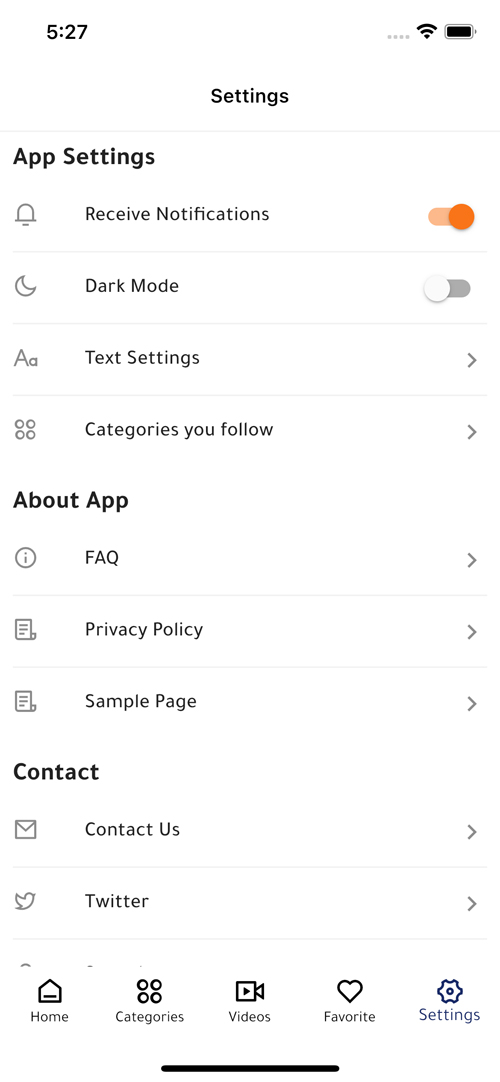The screenshot depicts a smartphone screen at 5:27, with full signal strength and battery life displayed on the top right corner. The interface showcases the settings menu of what appears to be the WordPress app. 

The menu items are as follows:

1. **Settings**: The main header.
2. **App Settings**: Sub-header.

Under the **App Settings** section:
- **Receive Notifications**: An option to receive notifications, indicated by a bell icon, which is turned on (highlighted in orange).
- **Dark Mode**: Control for dark mode, represented by a moon icon, which is currently turned off.
- **Text Settings**: Adjustments for text size, depicted with a large 'A' and a small 'A'.
- **Categories You Follow**: Indicates user preferences in categories, shown with four small dots icon.

Under the **About App** section:
- **FAQ**: Frequently Asked Questions, symbolized by an information icon (a small 'i' in a circle).
- **Privacy Policy**: Linked to the privacy policy document, represented by a document icon.
- **Sample Page**: Possibly a template or example page.
- **Contact Us**: Contact information or support, depicted by an envelope icon.
- **Twitter**: A quick link to the WordPress Twitter handle, shown with the Twitter bird icon.

At the bottom of the screen are navigation buttons:
- **Home**
- **Categories**
- **Videos**
- **Favorites**
- **Settings**

Each option is paired with a corresponding icon for easy identification. The interface is predominantly text-based, making it clear and functional for managing blog settings on the WordPress app.